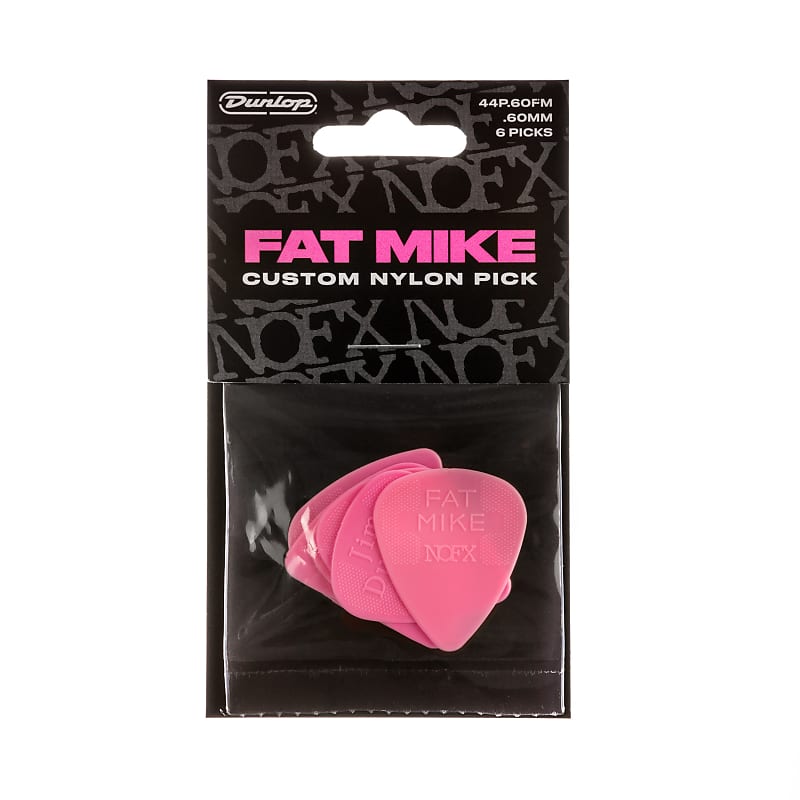The image depicts a retail package for Dunlop Fat Mike custom nylon guitar picks. The package is characterized by its black cardboard backing adorned with various texts and a clear plastic bag stapled to the lower half, containing six pink picks. At the top left of the card, "Dunlop" is prominently displayed, while the top right features the technical details: "44P.60FM.60mm 6 Picks." The middle section of the card highlights the name "Fat Mike" in bold pink letters, followed by "Custom Nylon Picks" in white letters. Each pick, visible through the clear plastic, showcases the "Fat Mike NOFX" branding. The package design incorporates a hole at the top, allowing it to be hung for display, suggesting it is meant for retail sale, likely on a website or in a music store.